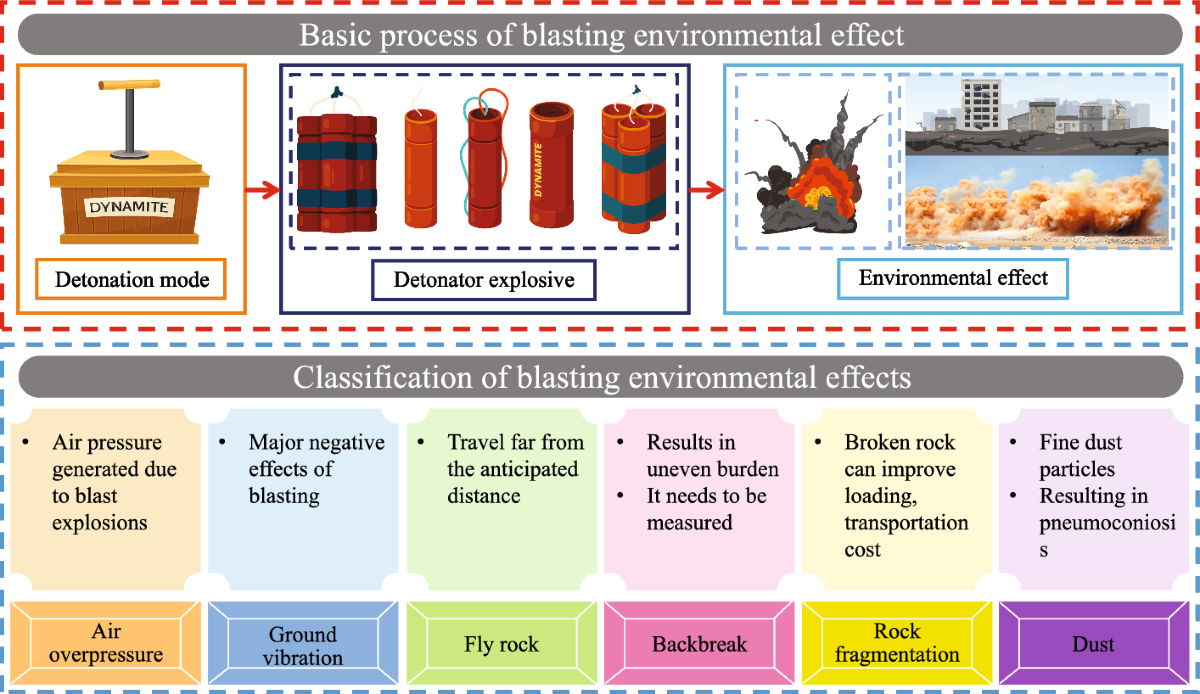The image is a detailed, multicolored diagram on a white background, framed by a red and blue dashed line. At the top, the title "Basic Process of Blasting Environmental Effects" is prominently displayed in white lettering against a gray background. The diagram features a sequence starting from a drawing of a wooden dynamite plunger labeled "Dynamite," alongside the text "Detonation Mode." An arrow points rightwards to a box labeled "Detonator Explosive," illustrated with images of bombs and dynamite. Further to the right, another arrow points to "Environmental Effects," depicted with images of explosions around a cityscape.

Beneath these illustrations, the diagram delves into the "Classification of Blasting Environmental Effects" with six color-coded rectangles, each highlighting a different impact:
1. **Air Overpressure** (orange): Air pressure generated due to blast explosions.
2. **Ground Vibration** (blue): Major negative effect of blasting.
3. **Fly Rock** (green): Rocks traveling far from the anticipated distance.
4. **Back Break** (pink): Resulting in uneven burden, which needs to be measured.
5. **Rock Fragmentation** (yellow): Broken rock that can improve loading and transportation cost.
6. **Dust** (purple): Fine dust particles that result in pneumoconiosis.

Each rectangle is distinctly colored—orange, blue, green, pink, yellow, and purple—and features black text, effectively categorizing and explaining the various environmental effects of blasting.